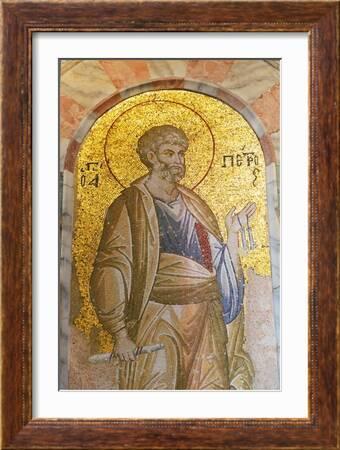The image is an old-style, framed painting housed in a vertical rectangular wooden frame, surrounded by a white background. The subject of the painting is a light-skinned, blonde man with a full head of hair and a thick beard, including a small goatee. He is depicted standing beneath an archway with an intricate Greek design, accentuated by a shimmering gold background. The man is dressed in an elaborate golden garment, reminiscent of contemporary loungewear but detailed and ornate. He wears a long gold jacket, bright golden trousers, and a vest-like undergarment that is blue with slight red accents on the side. A semicircle in red perfectly frames his head. In his right hand, he holds a parchment or scroll, and bandages or some additional object are in his left hand. Very small Greek text flanks him on the left and right edges of the painting.